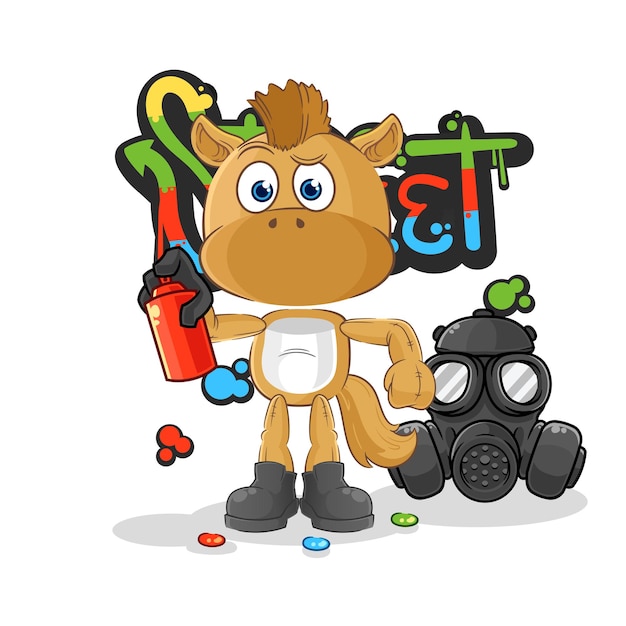The image depicts a cartoon character that seems to be a cow, although it has some features reminiscent of a horse, like a mohawk. The character is predominantly brown except for the belly and chest, which are white. It is wearing black boots and a black glove on its right hand, while holding a red spray paint can. The scene takes place on a white background, emphasizing the colorful details. Next to the character, on the right, lies a black gas mask with green paint on it. Beneath the character, there are three bean-shaped splatters of green, blue, and red paint. Behind the character, vibrant graffiti formed from yellow, green, blue, and red paints is visible, possibly spelling out "street," though the character partially obstructs this detail. This artistic image suggests the character has been engaging in graffiti art.